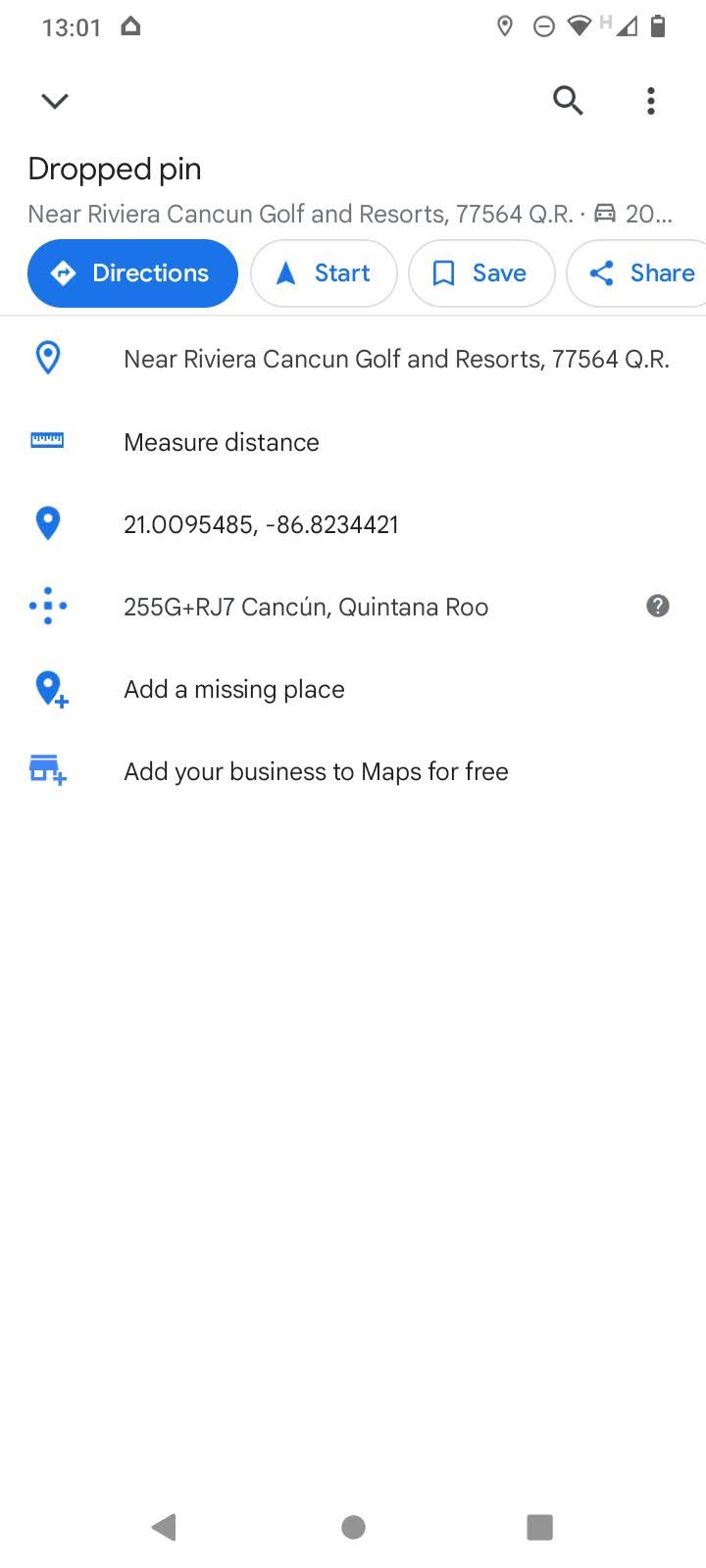Screenshot of a smartphone displaying mapping application at 13:01. The device shows an internet connection with one bar and a battery level at approximately 75%. The application's interface features a text box or search bar with a magnifying glass icon and a three-dot drop-down menu on an all-white background.

A prominent header reads, "Dropped Pin Near Riviera Cancun Golf & Resorts 77564QR20." Below this header are four actionable buttons: "Directions," "Start," "Save," and "Share."

The subsequent entries include:
1. "Near Riviera Cancun Golf & Resorts 77564QR" 
2. An instruction to "Measure Distance" accompanied by a ruler icon.
3. GPS coordinates: "21.0095485, -86.8234421."
4. An address code: "255G+RJ7 Cancun Quintana Roo."
5. Options to "Add a Missing Place" and "Add Your Business to Maps for Free."

The interface is designed to provide users with navigational and informational tools related to the selected pin location near the Riviera Cancun Golf & Resorts.